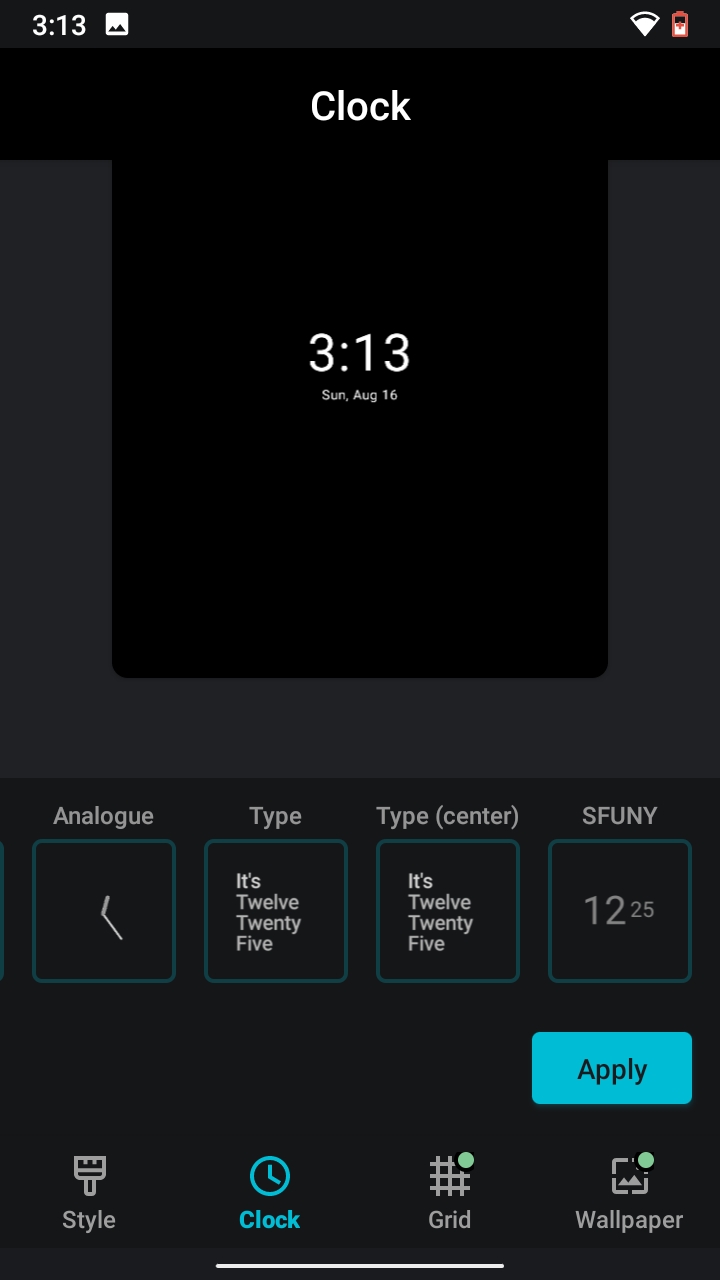This is a detailed screenshot captured from a smartphone at 3:13. The top left corner displays the current time, while the top right corner shows a nearly depleted battery, with less than a quarter remaining. The center of the top section is labeled "Clock." 

In the middle of the screen, large white numbers display the time as 3:13, accompanied by a smaller, barely legible date that reads "Sunday, August 14th."

At the bottom of the screen, there are several boxes with different labels just above them. From left to right, the labels are: "Analog," "Type," "Type Center," and "Spoony" or "Spunny." Below the "Analog" label, there's an image resembling a clock face with one hand pointing upwards and the other at a 45-degree angle. Below the "Type," "Type Center," and "Spoony" or "Spunny" labels, the time is consistently shown as 12:25.

These various sections likely represent different ways to display the time on the clock, offering alternative visual options for users who may prefer different formats or who have difficulty reading standard numeric representations.